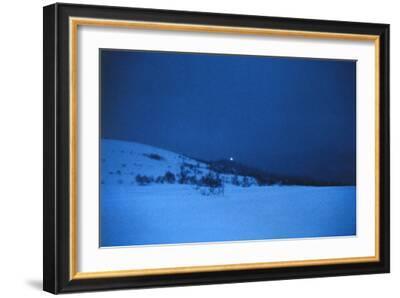This photograph features a rectangular photo frame with a sleek black border accented by a thin line of gold trim. Enclosed within the frame is a captivating piece of artwork depicting an outdoor snow-covered landscape. The scene captures an evening setting under a medium to dark blue sky. In the foreground, snow-blanketed hills gently rise and fall, leading the eye towards a cluster of distant trees. A dark peak looms farther back, adding depth to the scene. A small illuminated light punctuates the serene, wintry landscape, casting a subtle glow that contrasts beautifully with the surrounding darkness. The artwork is neatly bordered by a clean white mat. Behind the frame, a faint shadow is cast onto the backdrop, which is a plain white surface, adding a touch of dimension to the presentation.